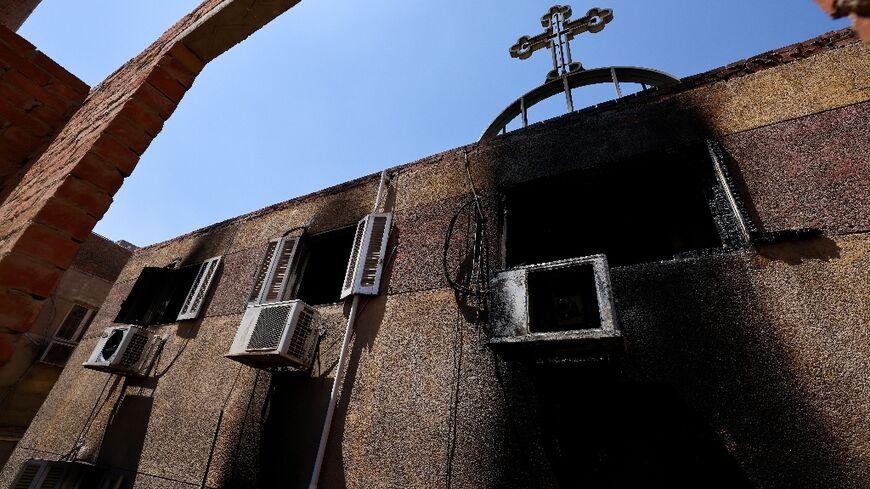The image depicts the side of a brown and black building, likely an abandoned church, as indicated by a prominent cross mounted on the roof. The photograph, taken from ground level during the daytime, shows a clear blue sky above. The building's facade features three windows, each fitted with air conditioning units, and extensive black soot covering parts of the walls and air conditioners, suggesting a past fire incident. 

A distinctive red brick structure is visible in the upper left corner, adding texture and contrast to the brown, soot-streaked concrete walls. One window has shutters attached, and an arch extends from the lower left to the top center, where it disappears beyond the photo's border. There is also a small gate visible, enhancing the detailed view of this weathered, yet historically rich, building.